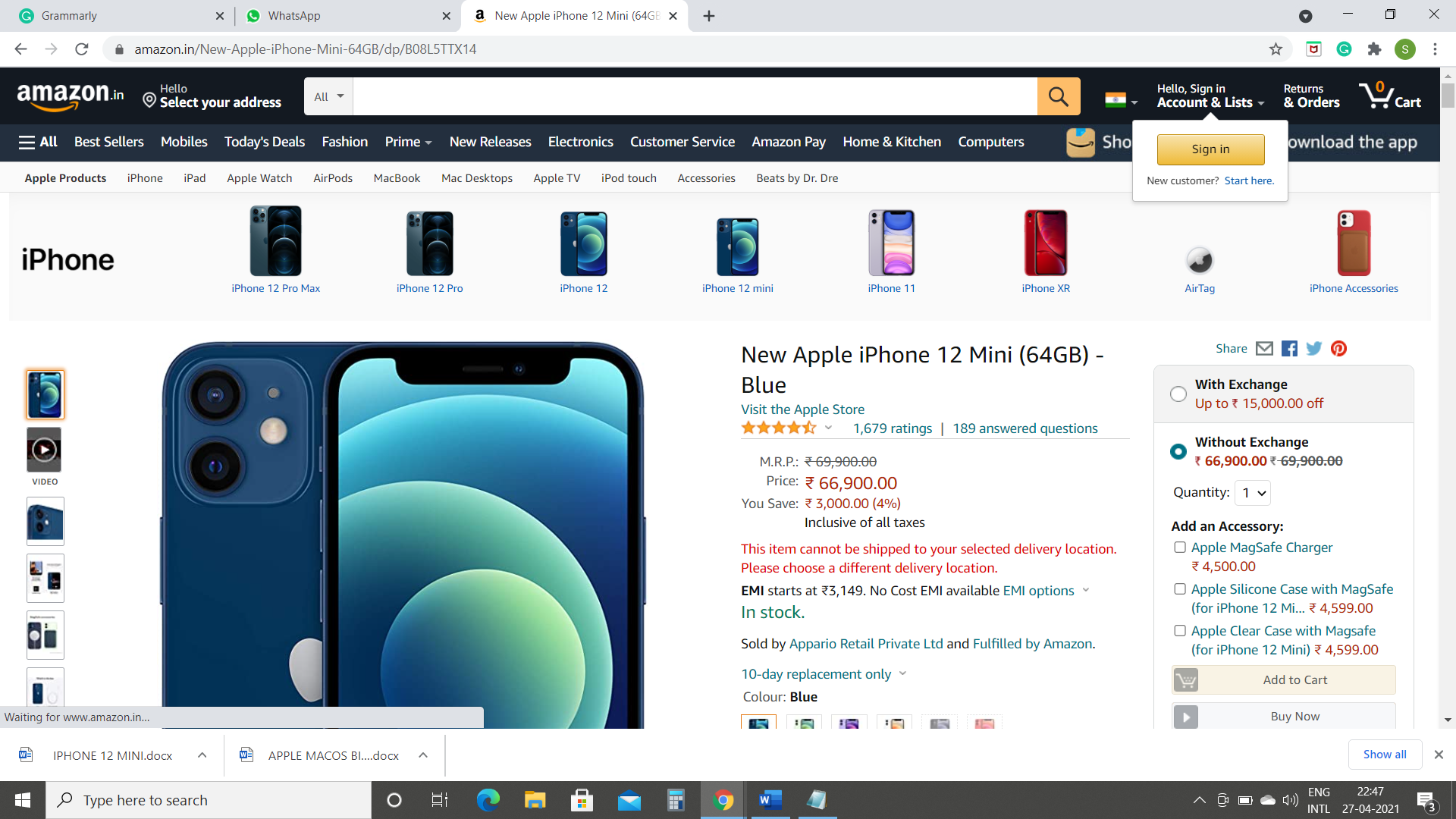This screenshot from an Amazon page displays the product listing for a new Apple iPhone 12 Mini in a 64GB blue variant. The browser also has WhatsApp and Grammarly tabs open. At the top of the Amazon page, the logo is visible along with options to select your address, a search bar, and other navigation elements written in Spanish, suggesting a Mexican market version of the site. The page greets users with a "Hello, sign in" prompt for accounts and lists, alongside options for new customers to start here, view orders, and see the cart, currently showing zero items. 

The focus is on the phone, a new Apple iPhone 12 Mini, which has accumulated 1,679 customer ratings averaging four and a half stars, and has 189 answered questions. The marked retail price is listed as MXN 69,900.00, but it is currently available for MXN 66,900.00, saving customers MXN 3,000, or 4%, inclusive of all tax. However, this item cannot be shipped to the selected delivery location, and customers are prompted to choose a different address. The product also offers EMI (Equated Monthly Installment) options starting at MXN 3,149 with no cost EMI available. The phone is in stock and sold by Appario Retail Private Ltd.